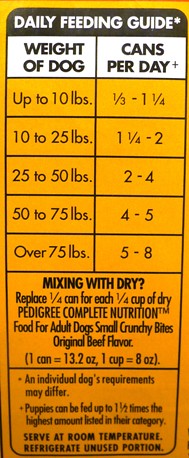This image is an extreme close-up of a section of a dog food bag. The upper part of the image prominently features the Daily Feeding Guide printed in brown text. Below this title, there are white squares that provide feeding instructions based on the dog's weight, indicating the number of cans to be fed per day. The guidelines are as follows: 

- For dogs up to 10 pounds, feed 1/3 to 1 1/4 cans per day.
- For dogs weighing 10 to 25 pounds, feed 1 1/4 to 2 cans per day.
- For dogs weighing 25 to 50 pounds, feed 2 to 4 cans per day.
- For dogs weighing 50 to 75 pounds, feed 4 to 5 cans per day.
- For dogs over 75 pounds, feed 5 to 8 cans per day.

Additionally, there are mixing instructions printed in a yellowish-orange color, advising to replace 1/4 can for each 1/4 cup of dry food when mixing with dry kibble. The product is "Pedigree Complete Nutrition for Adult Dogs" and the flavor specified is "Original Beef Flavor."